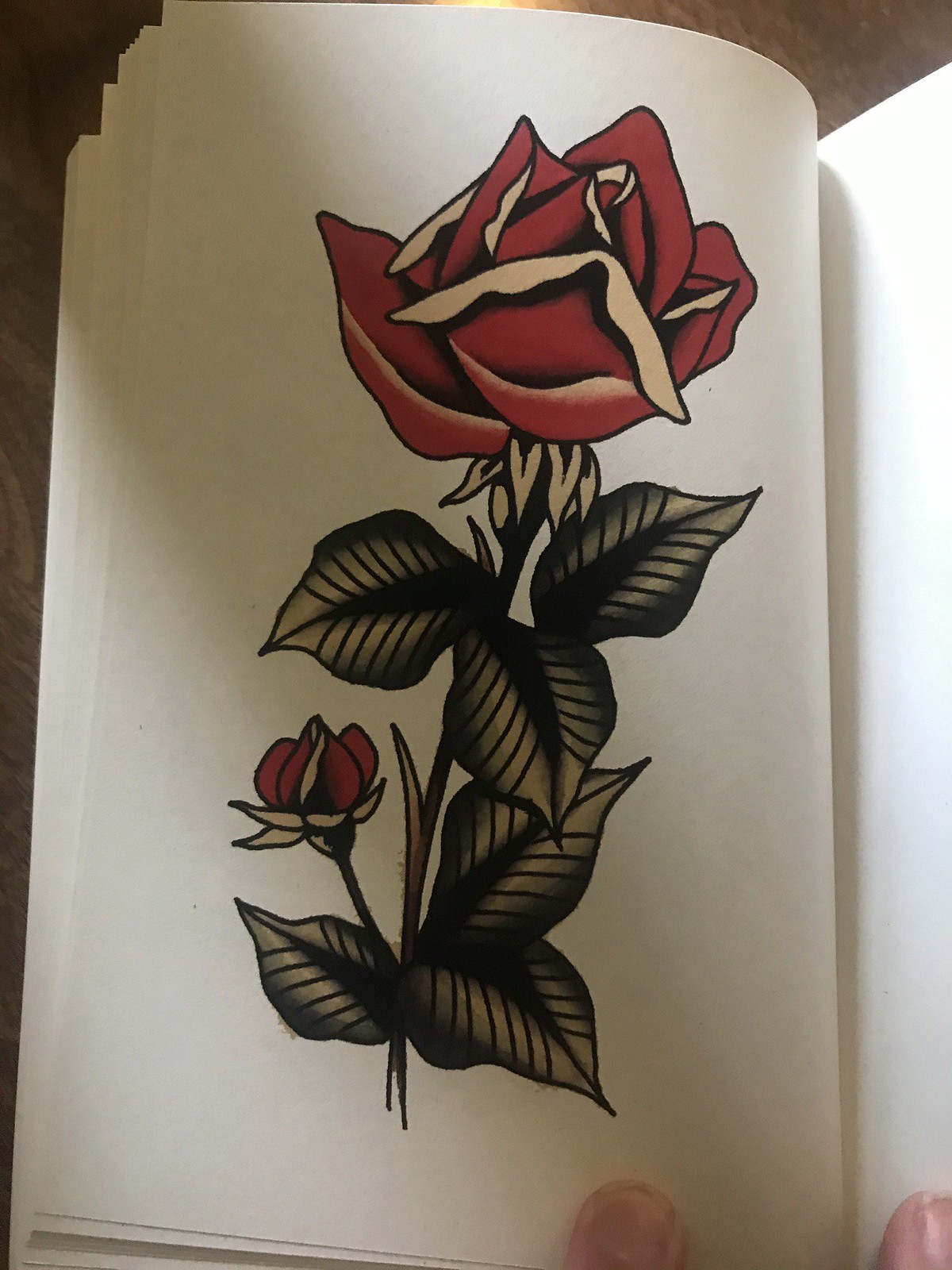The image depicts a drawing in a bound white notebook lying open on what appears to be a dark wooden table surface. The drawing itself features a detailed depiction of a red rose at the top of the page, with a green stem running vertically through the center. Attached to this main stem is a smaller red rose bud located in the bottom-left quadrant of the page. There are six green leaves positioned strategically—three below the larger rose and three below the smaller bud. The artwork employs a distinct American style characterized by pronounced lines and solid, harsh shadows. In the bottom-right corner of the image, two Caucasian fingers—likely the middle and ring fingers—are seen holding the page open, preventing the notebook from closing.